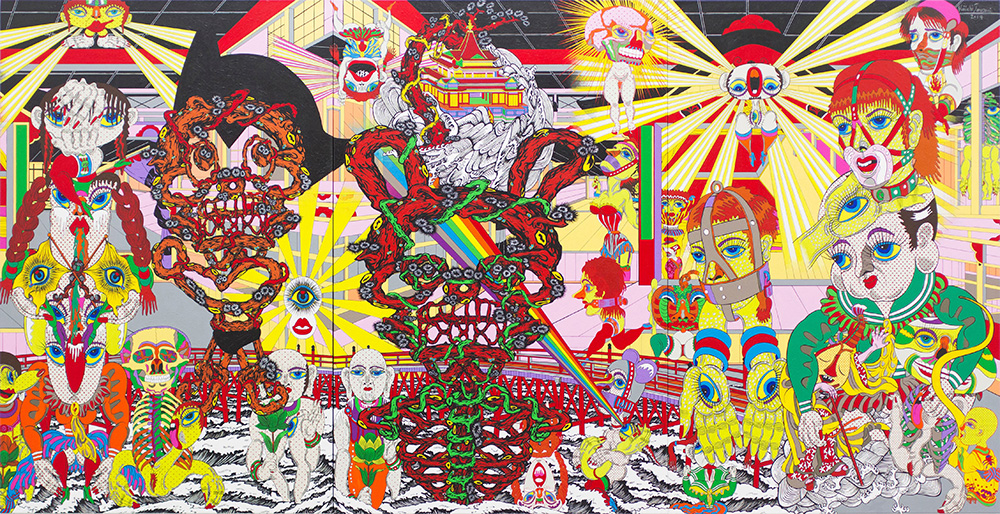The painting is a vibrant, surreal, and somewhat abstract composition filled with an array of diverse figures and vivid colors. Dominating the right side are yellow, sun-ray-like beams emanating from a clownish face with blue eyes and a red nose, which could be mistaken for a mouth. Emerging from these rays are an assortment of characters, including disembodied human legs with a skull that still possesses eyes and a brain, a figure wearing a red helmet and a face mask, and a woman with red hair adorned with leather straps around her mouth and forehead.

Among the colorful chaos, yellow hands with eyes can be seen interspersed, adding a sense of mystical or religious undertone. Skulls appear multiple times throughout, contributing to the eerie collage of figures. Two heads on the far right stand out: the lower one resembling a Buddha with a green headdress, and an upper head adorned with yellow and pinkish hues and red stripes on its face. The whole image is washed in an intense palette of reds, yellows, blues, greens, and purples, with countless eyes scattered across the figures, suggesting an Asian artistic influence. Additionally, a rainbow arches through the middle of the scene, cutting through some beams of light that stream across the painting. The mix of tall and short characters, some with ancient features like stretched ears, adds to the rich and complex visual narrative.